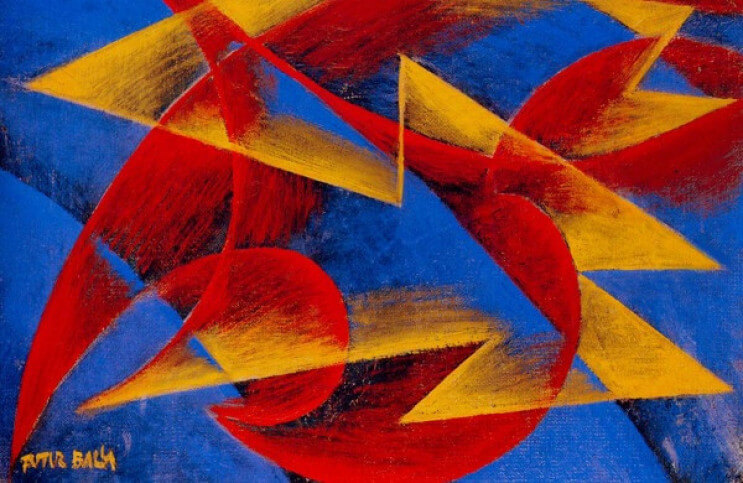In this abstract painting, vibrant hues and dynamic shapes dominate the canvas. The background is primarily blue, featuring wavy, rounded shapes that flow from the left diagonally downwards to the right. Interspersed throughout the composition are vivid oranges, reds, and yellows creating an energetic and chaotic pattern. The orange elements resemble sideways triangles, while the red features transition between swirling, spiky curves and pointed triangular forms. Yellow accents, sharp and jagged like lightning bolts, contribute to the painting's electric feel. A barely legible yellow signature, presumably the artist’s, is located in the bottom left corner. Despite its chaotic appearance, the piece plays with color and shape in a captivating and intricate manner.